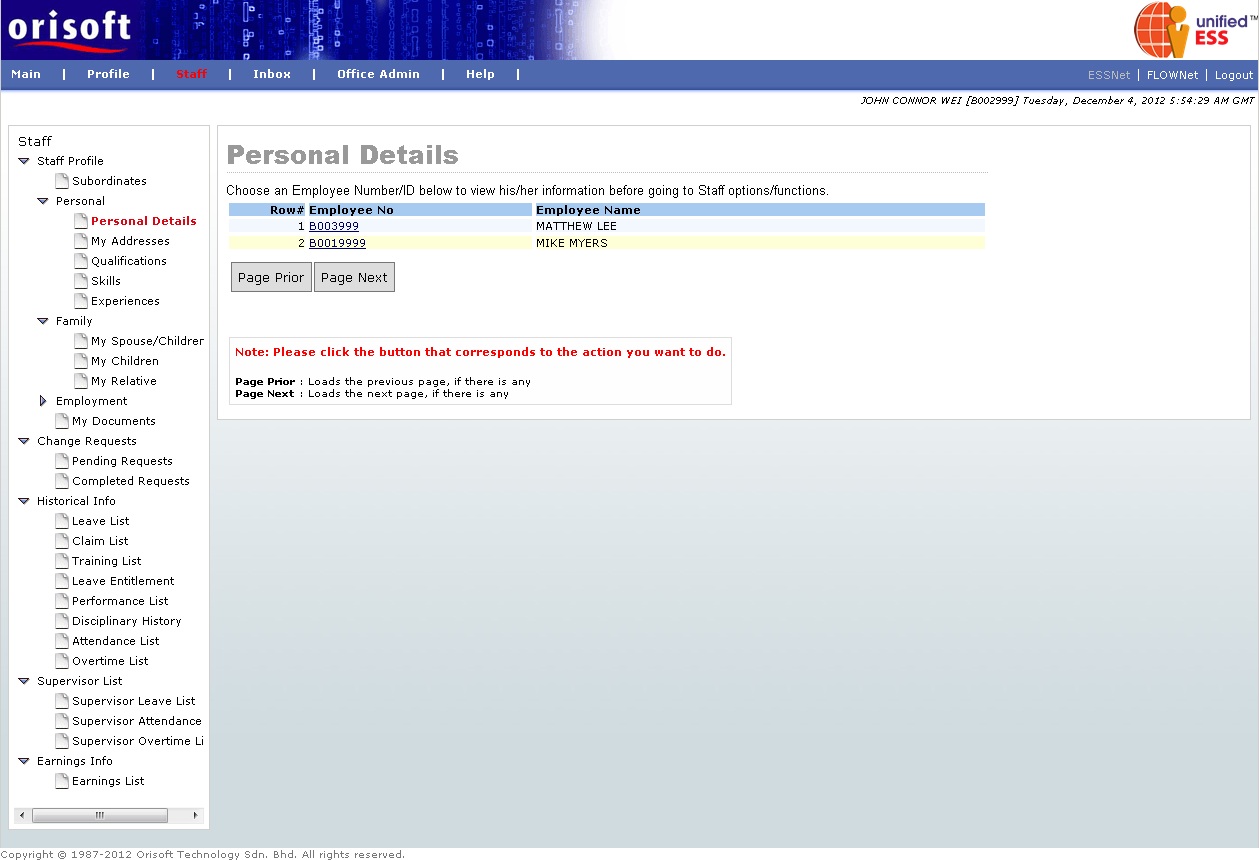The image displays a computer interface, prominently featuring a gradient background that transitions from dark blue at the top to white towards the center. At the top, the text "Aura Soft" is displayed in white letters, underlined by a red line. In the backdrop, there are faded images of trees blending seamlessly into the background.

On the right-hand side, a small red globe icon is visible alongside the text "Unified ES," with a stylized letter "D" featuring a dot above it. Below this, a blue box houses various headings in white text, including "Beats," "Profiles," "Inbox," "Office Admin," and "Help," with each section likely corresponding to different functional areas of the software.

Lower on the right side, a flowchart icon and a logout button are present. Meanwhile, on the left side, there is a white box listing several options such as "Staff," "Staff Profiles," "Personal and Family," "Employment Change Requests," "Historical Info," "Supervisor List," "Earnings Info," each accompanied by a small green arrow indicating expandable sections. A gray toggle button is situated at the bottom of this list.

Adjacent to this, the main display area contains a large white box. At the top of this box, the heading "Personal Details" is displayed, followed by a blue dotted line. Beneath it, the instruction reads: "Choose an employee number/ID below to view his or her information before going to staff options and functions."

Further down, there are three colored strips—blue, light blue, and yellow—each labeled with "REW," "Employee Number," and "Employee Name" respectively. Listed employees include Matthew Lee and Mike Myers. Below the list, two gray navigation buttons labeled "Page Prior" and "Page Next" allow users to traverse through different pages of employee information.

At the very bottom, there is another white box containing red text instructions that state: "Note: Please click the button that corresponds to the action you want to do. 'Page Prior' loads the previous page if there is any, and 'Page Next' loads the next page if there is any." The image concludes with a large gray box at the bottom of the interface.